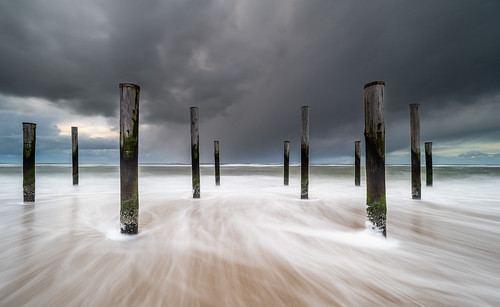The photograph appears to be an artistic depiction, capturing a desolate and dramatic scene. The foreground features old wooden pilings, remnants of a former pier, emerging from what might be the frozen surface of a lake or an icy shoreline. The pilings are arranged in a particular pattern: two aligned in a row on the left, followed by three rows of pilings to the right, each with three pilings, and then progressing to two and finally a single piling most rightward. The surface appears shiny, reminiscent of a frozen lake undergoing a storm, with wisps of snow or mist skittering across its surface in linear, fog-like streaks. The top part of the pilings remains visibly wooden, while their bases show signs of being worn by water or ice.

In the background, the sky is a dark, foreboding gray with low-hanging clouds, adding to the sense of an impending storm. The horizon hints at a slightly bluish-gray tone, contrasting eerily with the near-black storm clouds above. Beneath the pilings, a sand-colored ground or ice is visible, further accentuating the cold, harsh atmosphere of the scene. Together, these elements create a haunting and ethereal image, blurring the lines between reality and imaginative art.